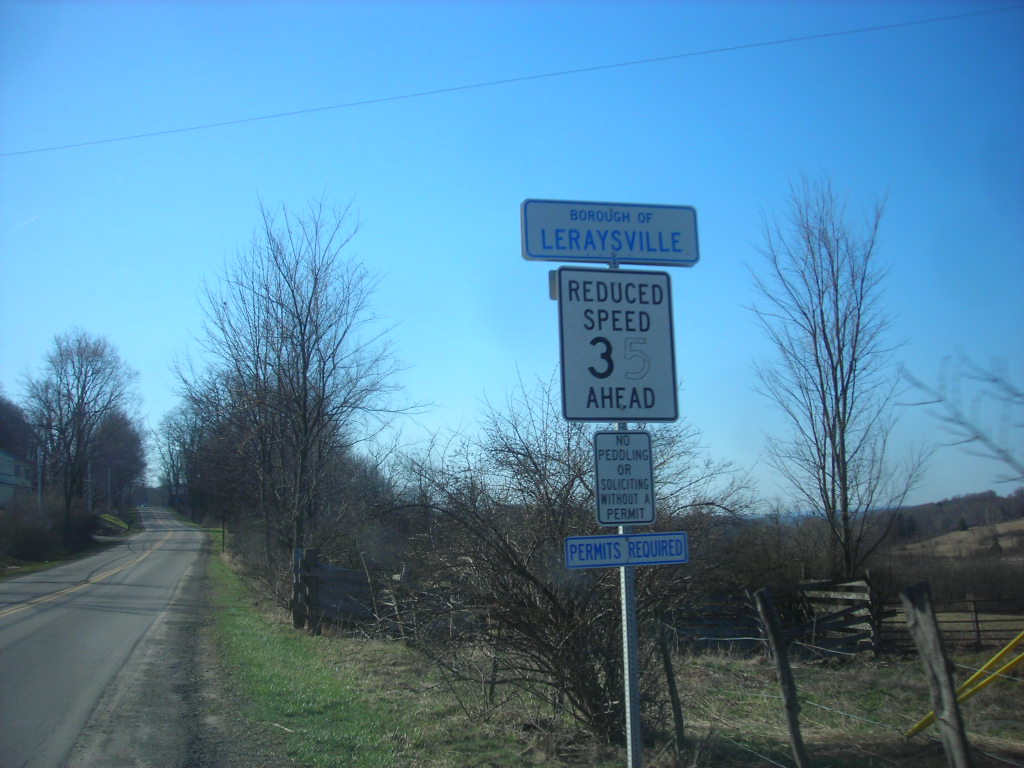This photograph captures a series of signs posted alongside a long, uphill road. The road curves to the left, with the photographer positioned in a lush, green grassy area adjacent to it. The scene suggests a wintry or late fall setting, as leafless trees are visible along the brown wooden fence down the street and nearby. 

The top sign is white with blue lettering, reading "Borough of Laraisville." Below it, a white sign with black lettering states "Reduced Speed 35 Ahead." Notably, the number '5' is merely outlined, having lost its black fill. Further down, another white sign with black lettering warns, "No Pedaling or Soliciting Without a Permit." At the bottom, a final white sign with blue lettering declares, "Permits Required."